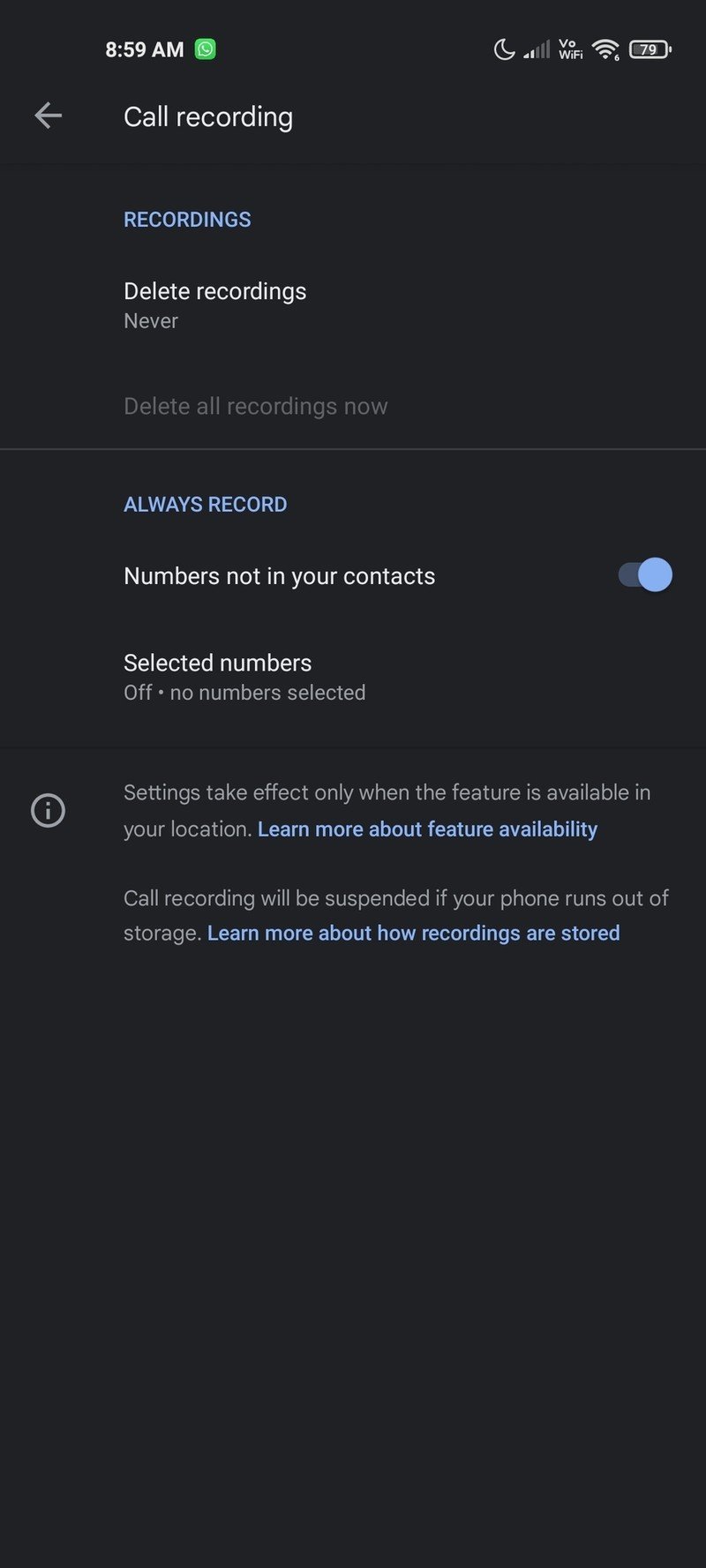### Detailed Caption for the Image

The image is a screenshot of a website displayed on a cell phone, with a predominantly black background. In the upper left-hand corner, the time is shown in white print as "8:59 AM." Next to the time, there is a small, green square with rounded corners, containing a white cell phone icon inside. Moving to the right side of the upper area, there are icons indicating a crescent moon (Do Not Disturb mode), cell signal strength, Wi-Fi signal strength, and "VO Wi-Fi." The battery level is displayed at 79%.

Below this status bar, there is a leftward-pointing arrow and the label "Call Recording" with a capital C. Underneath this heading, there is text in blue, all in capital letters, that says "RECORDINGS." Following this, the options "Delete recordings" and "Never" are displayed, along with a faded option that reads "Delete all recordings now."

Further down, the section titled "ALWAYS RECORD" in the same blue, all-caps print follows, with the subtext "Number is not in your contact" turned on, and "Selected numbers off," indicating no numbers are selected.

At the bottom, there is an informational message indicated by a circle with an 'i' inside, reading: "Settings take effect only when the feature is available in your location." Below this message, there is a blue hyperlink text "Learn more about feature availability." Another informational note states: "Call recording will be suspended if your call runs out of storage." Lastly, there is a blue hyperlink saying "Learn more about how recordings are stored."